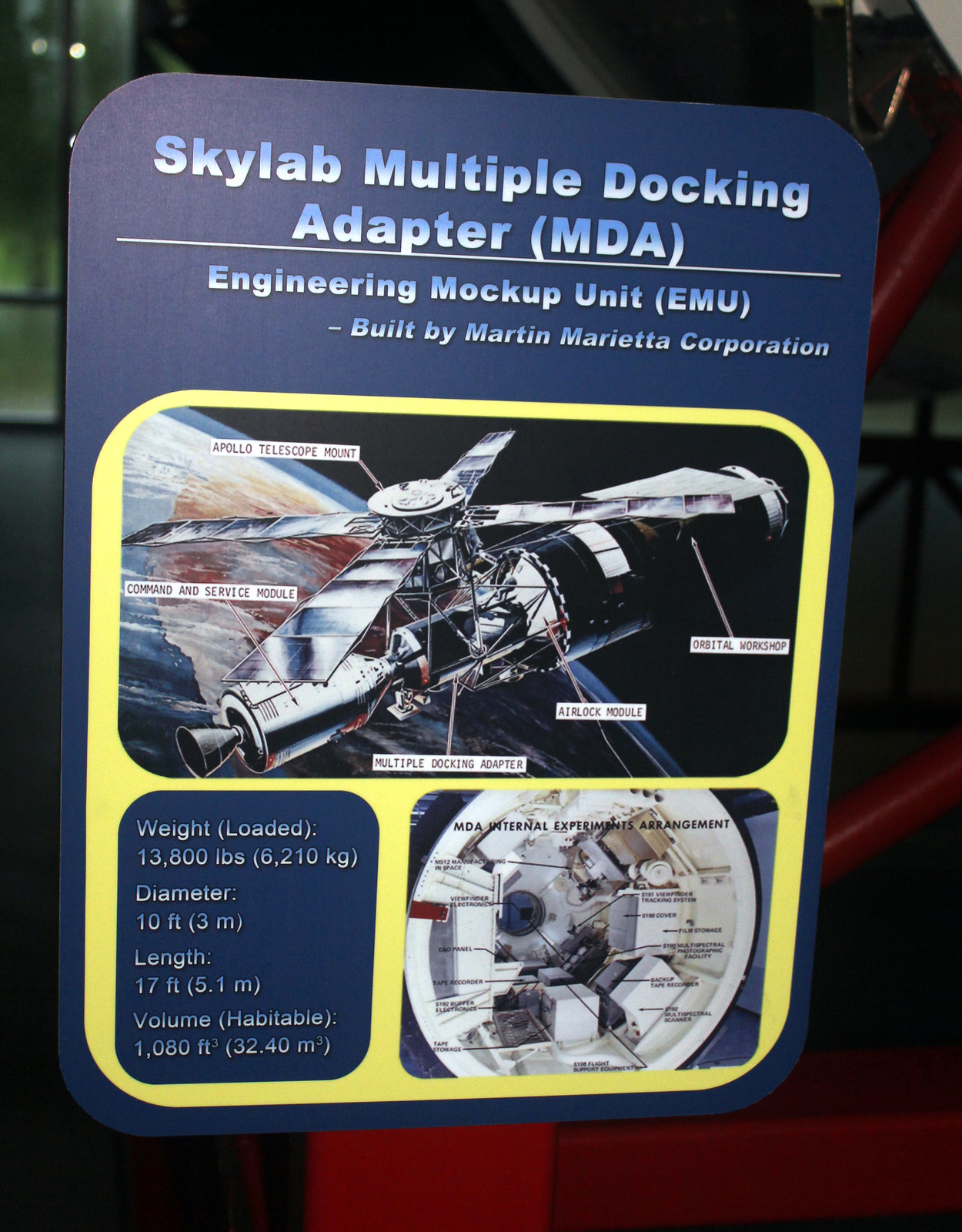The infographic, likely displayed in an aerospace museum, provides a detailed overview of the Skylab Multiple Docking Adapter (MDA). Against a steely dark blue background, the top section features a fading light blue to white text that reads "Skylab Multiple Docking Adapter (MDA)" and "Engineering Mockup Unit (EMU) built by Martin Marietta Corporation." Below is a yellow square box showcasing three unique images. The top image illustrates the Skylab space station with labeled components: the Apollo Telescope Mount, Command and Service Module, Multiple Docking Adapter, Airlock Module, and Orbital Workshop. The bottom left graphic lists the technical specifications such as weight, diameter, length, and volume. To the bottom right, a photo details the interior of the MDA with lines indicating different parts of the module. The display is framed by a red metal structure, suggesting its setting within an educational exhibit or museum.